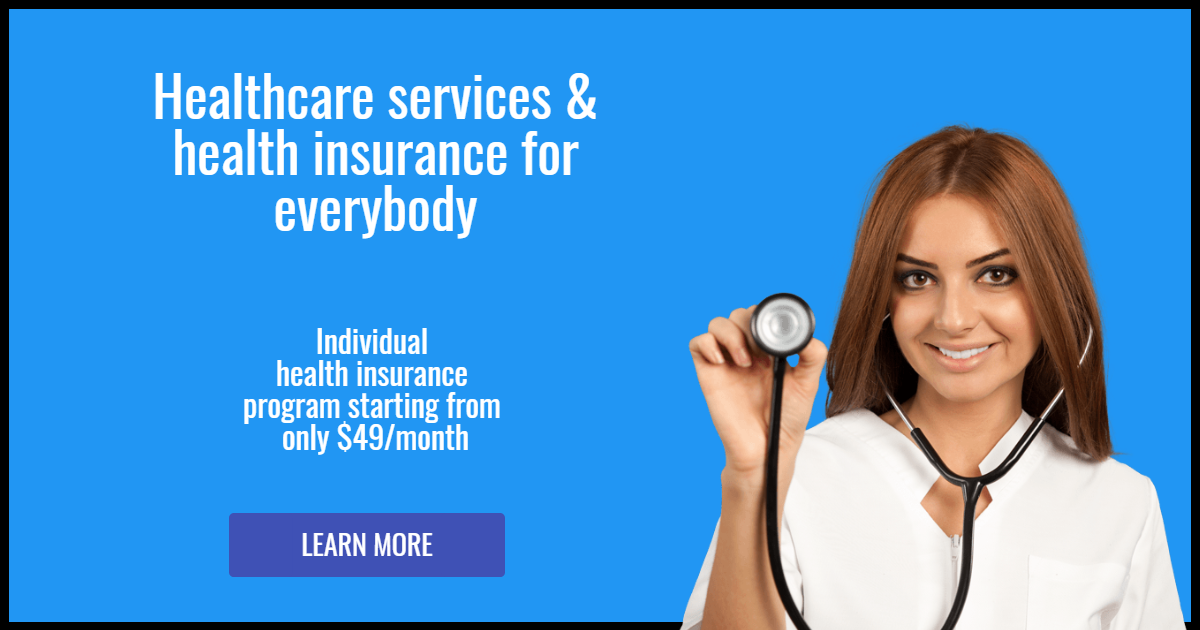The image is a screenshot from a web page with a sky blue background, bordered by a thin black line. In the lower right-hand corner, a photograph of a young woman, likely in her mid-20s and possibly of Latino descent, is superimposed on the background. She is smiling, with reddish-brown hair parted in the center, and is dressed in a white uniform with a stethoscope placed at her ears, holding the chest piece with her right hand.

On the left side of the image, there is a prominent headline in white font reading "Healthcare Services and Health Insurance for Everyone." Below the headline, a smaller white font text details, "Individual Health Insurance Plan, Health Insurance Program, starting from only $49 a month." Further down, a darker blue rectangle contains the white-text call-to-action, "Learn More."